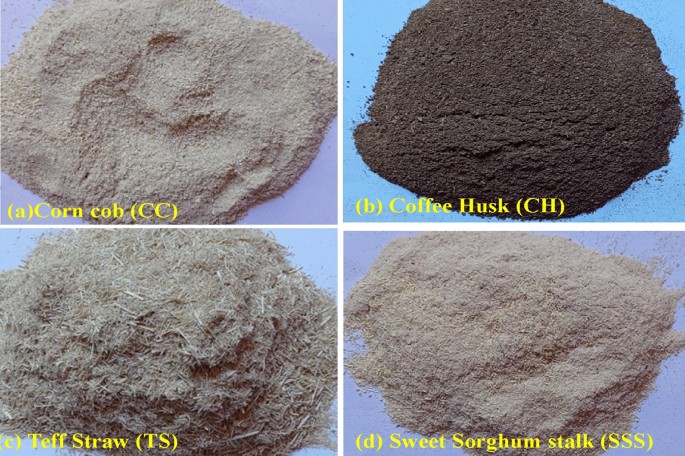This four-panel image showcases different types of plant-based powders, each set against distinct colored backgrounds. The top left panel, labeled 'A. Corn Cob CC,' features a fine grayish powder resting on a purplish background. To its right, the top right panel labeled 'B. Coffee Husk CH' displays a very fine, dark chocolate brown powder atop a blue surface. The bottom left panel, marked 'C. Teff Straw TS,' contains gray, stringy clumps resembling lawn scrapings against a blue background. Lastly, the bottom right panel identified as 'D. Sweet Sorghum Stock SSS' shows a fine beige powder placed on a purplish background. Each component is carefully labeled in yellow lettering.